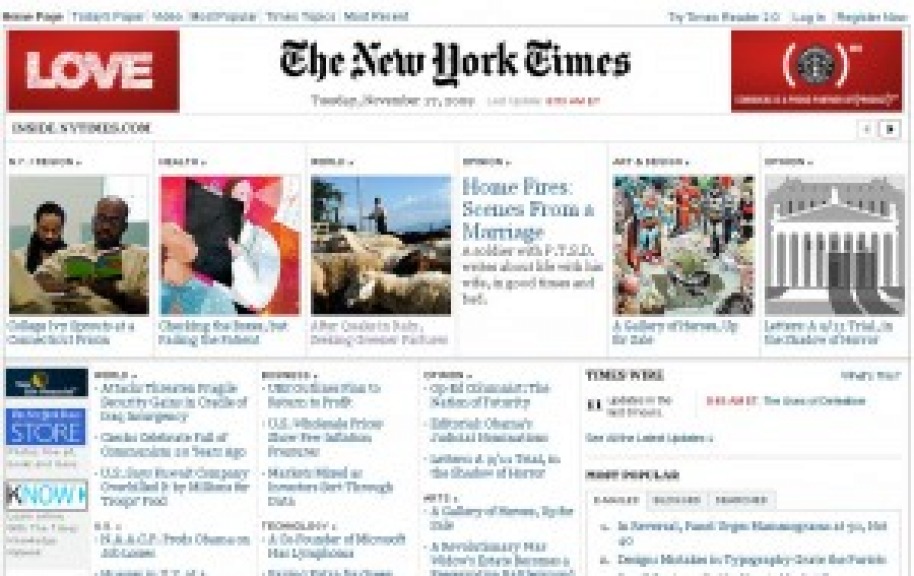The image depicts a blurred webpage of The New York Times. Prominently displayed in the center is "The New York Times" header. To the left, a striking icon with the word "LOVE" inside a red rectangular box stands out. Despite the overall blurriness of the image, which obscures 97% of the text:

1. The first story thumbnail features an image of what seems to be two jail inmates.
2. The second image is vibrant, predominantly pink, and resembles a quilt or patchwork.
3. The third depicts livestock, likely cows or sheep, with a person monitoring them.
4. The fourth image accompanies a headline with partially legible words that suggest themes of "home fires" and "marriage."
5. The fifth image remains indistinct due to the blur.
6. The sixth image appears to be a clip art figure, predominantly black and white, possibly depicting the White House or a similar monumental building.

At the bottom of the screen, various news links are barely visible, contributing to the overall blurred presentation of the webpage.